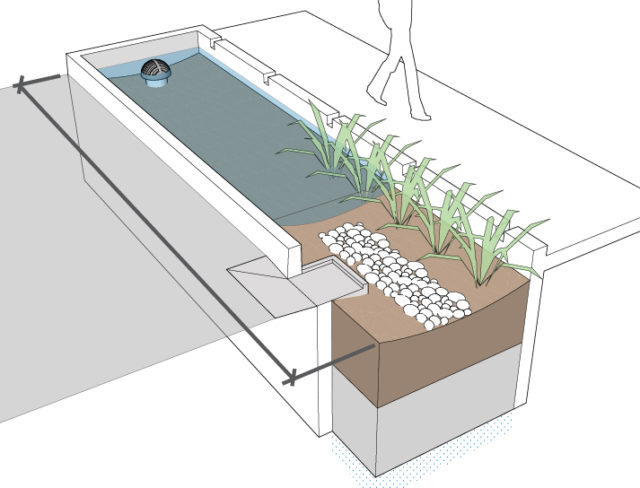The image is a detailed architectural drawing and 3D model showcasing a water drainage system integrated next to a sidewalk. The design features a section with plants that both absorb excess rainwater and facilitate drainage. The illustration includes a cutout of a box-like structure, allowing visibility of the internal components. Inside, there is a brown dirt layer interspersed with larger rocks for effective drainage. On one side of the box, water is depicted, though it's not completely filling the space. A drain pipe is visible, indicating how excess water would be managed. The scene also shows a person's legs walking on a white platform adjacent to the drainage area. The detailed elements, such as the gray clay, green plants, and the overall white background of the walkway and drawing, paint a comprehensive picture of a well-thought-out urban water management solution.